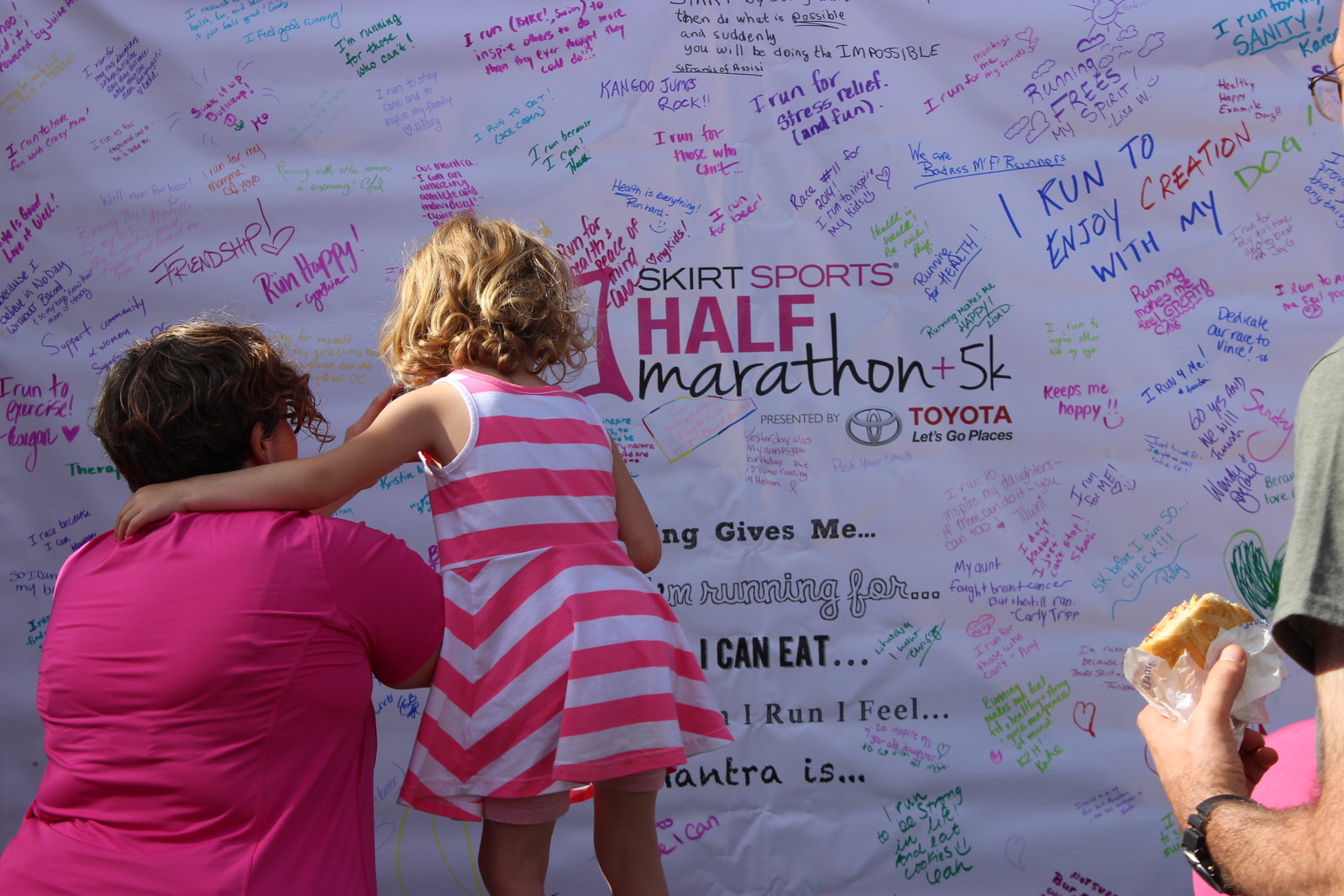In the image, a mother and her young daughter, approximately five to six years old with short blonde hair, stand with their backs to the camera as they sign a large, white banner covered in handwritten messages. The banner, titled "Skirt Sports Half Marathon and 5K," prominently features the Toyota logo with the slogan "Let's Go Places." Participants appear to be writing their reasons for running on the banner, with messages such as "I run for stress relief" and "I run to enjoy creation with my dog" visible among the notes. The mother, dressed in a pink shirt, and the daughter, in a white and pink striped dress, are focused on adding their contribution. To the right, a man in a green shirt and glasses watches while eating a sandwich. The scene conveys a community's support and personal motivations linked through the act of signing the banner.